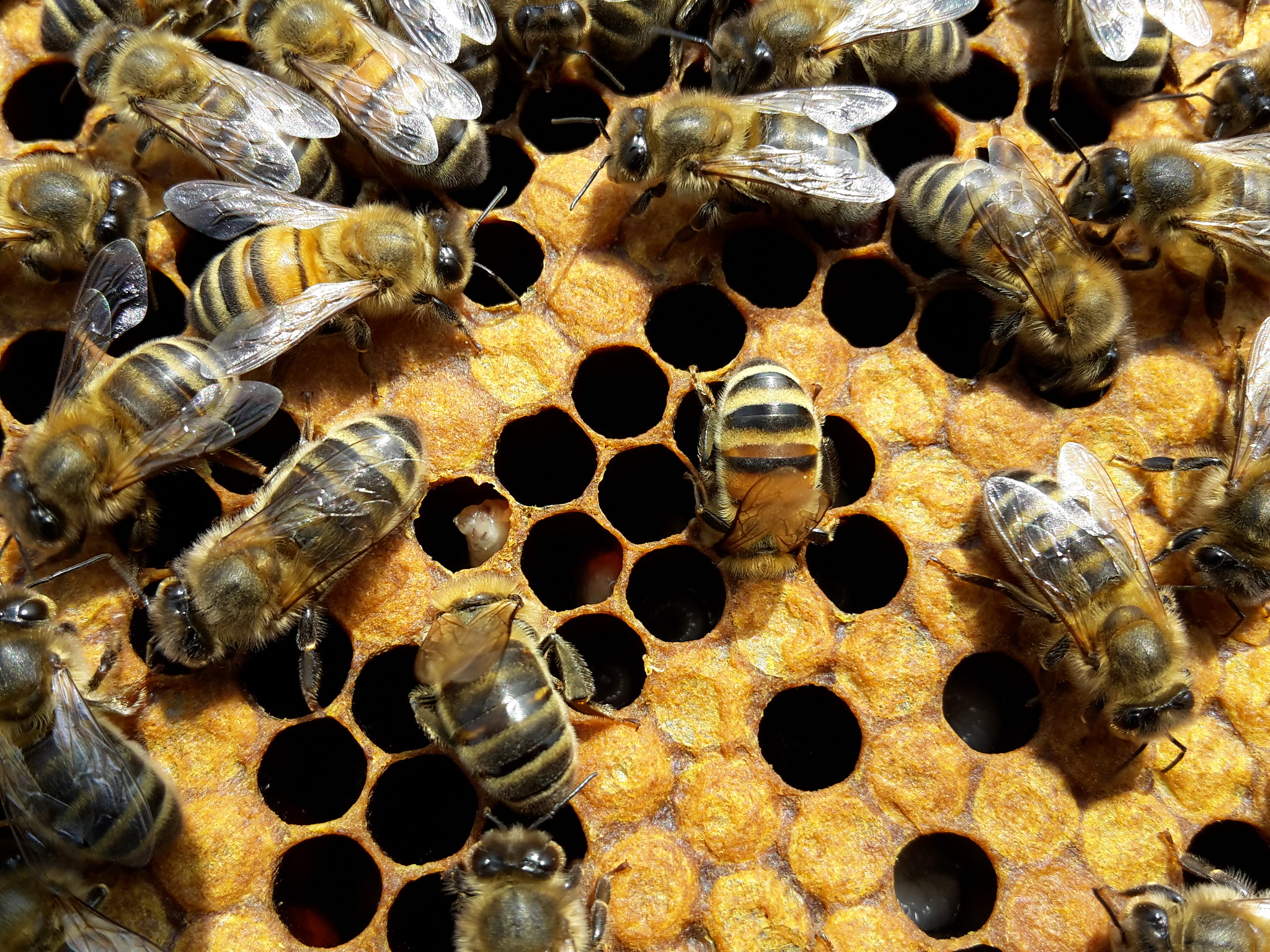This detailed, color photograph in landscape orientation captures a densely populated honeycomb surface teeming with approximately 25 honeybees. The bees are vividly colored with gold and black horizontal stripes, and their translucent silver wings are distinctly visible. Most bees are actively buzzing around, with a few partially inside the honeycomb cells. The hive itself features a mix of bright orange, yellow, and dark orange hues, interspersed with numerous open black circular cells, especially concentrated in the middle. The bees are spread across the top left and right sides of the image, while the central part predominantly showcases the honeycomb structure with some open sections scattered. The picture is a highly zoomed-in, realistic representation, focusing solely on the hive and its hardworking inhabitants, without any additional text or background context.